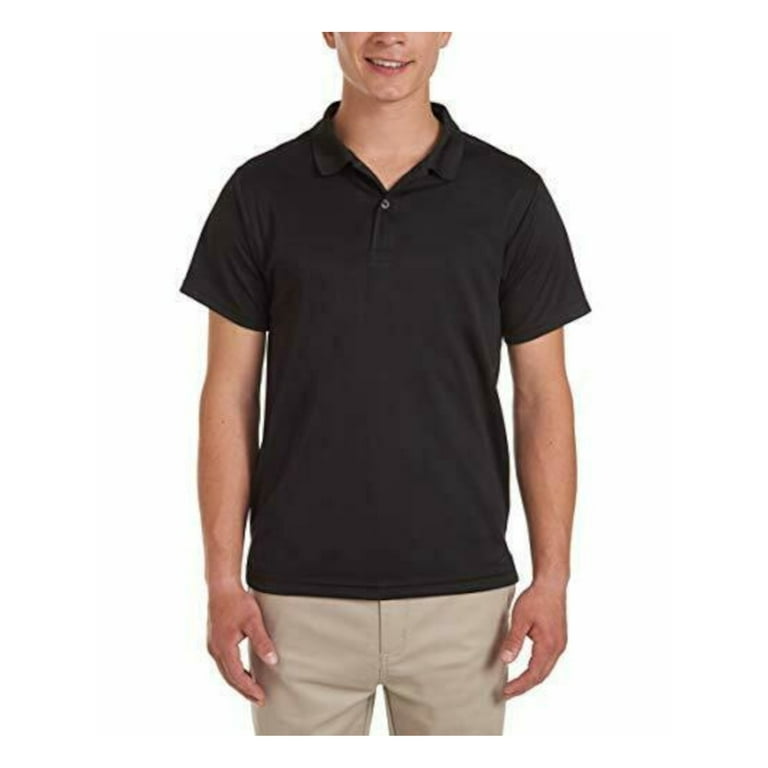This image features a man modeling a black polo shirt against a solid white background, likely intended for advertisement or retail purposes. The shirt, which is the focal point of the photograph, features a stylish three-button collar that is neatly folded over. It has short sleeves and is paired with khaki bottoms, adding a casual yet polished look. The man's pleasant smile is visible, although the top of his head and his legs are cropped out of the frame, further directing attention to the apparel. The seamless white backdrop ensures that the shirt stands out, making it an ideal candidate for promotional use.